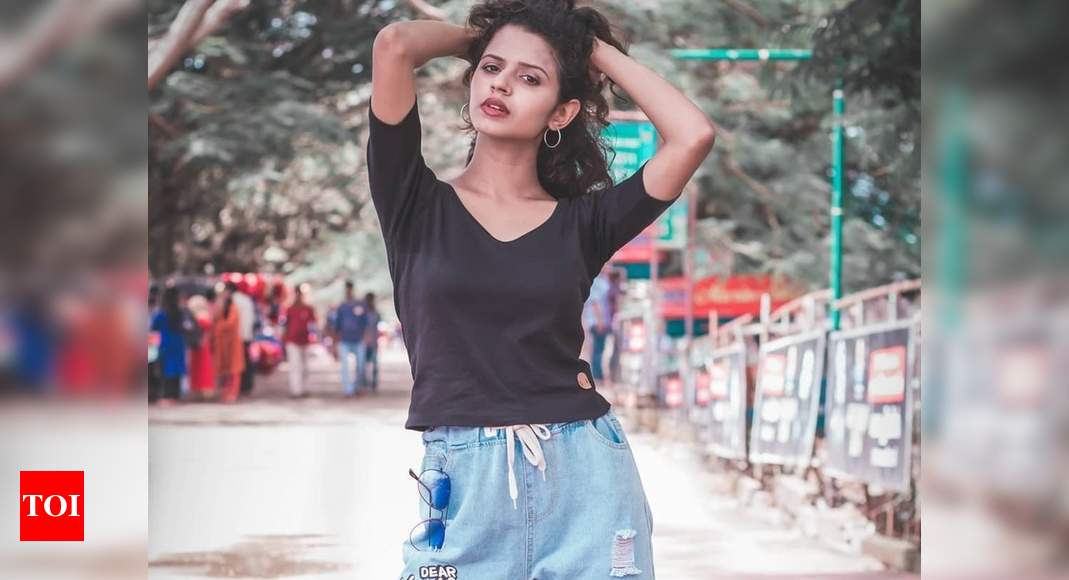The image is a detailed photograph of a young woman posing outdoors, centered against a blurred backdrop. The woman, who has dark hair styled up with her hands, is wearing a black three-fourths sleeve V-neck shirt and denim drawstring shorts. Aviator sunglasses with blue lenses dangle from her right pocket. She also sports hoop earrings. The background features a pathway enclosed by some sort of green fencing or barricades, with green signage that is difficult to decipher due to the blur. There are a few people walking in the distance, and the setting appears to be in a Spanish-speaking area, possibly in Mexico. At the bottom left of the image, there is a small red square with the text "T.O.I."